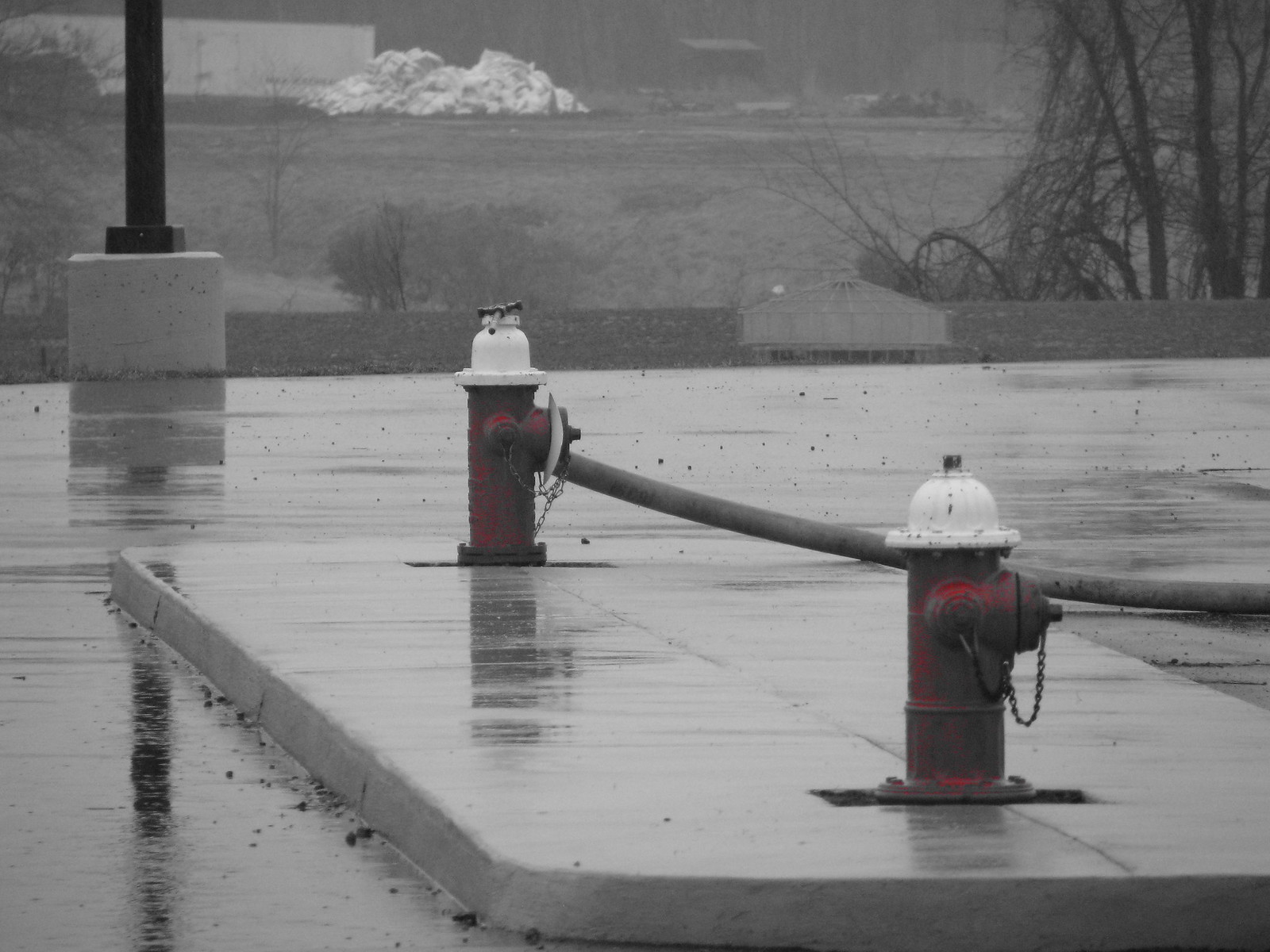In this photograph, taken on a rainy day, we see a vividly detailed scene dominated by two prominent red fire hydrants with white domes on top. They are positioned on a raised dark gray concrete curb in the center of a very wet road, with small reflective puddles scattered around. The hydrants are slightly marred with black splotches and dirt, and the one on the left has a large gray hose attached, extending off to the right edge of the image.

The scene behind the hydrants features a mix of elements. Towards the far end of the road, there's a street light mounted on a cylindrical concrete base, and next to it sits a large bench. The background appears somewhat monochromatic, potentially due to the overcast weather, with a faint pile of dirty white snow and leafless trees lining both sides of the road, suggesting a chilly, wintry atmosphere. Debris litters the wet pavement, enhancing the sense of desolation and cold characteristic of the setting. The composition of the photograph, with its play of colors and reflections, imparts an artistic, almost painterly quality to the image.